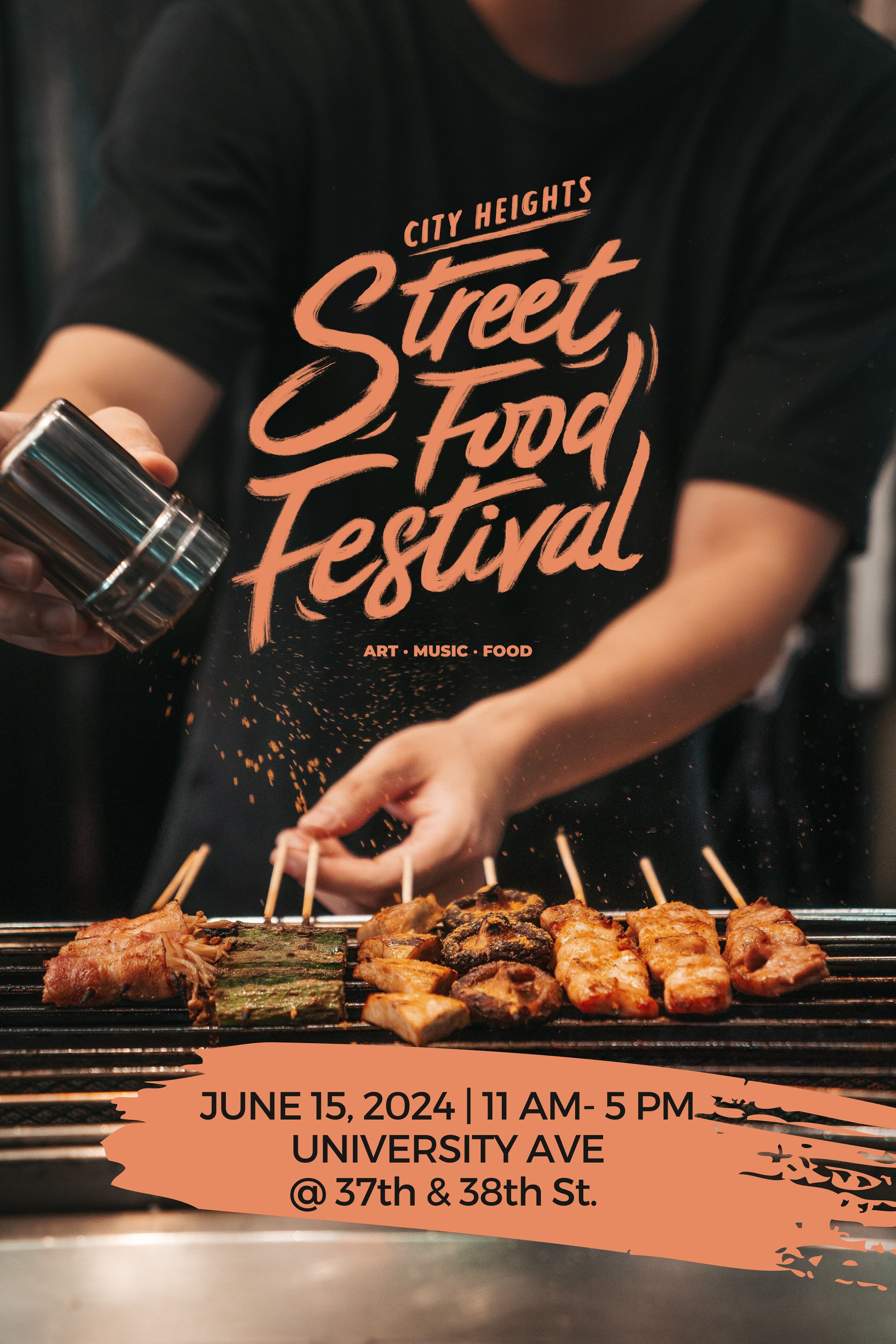The image shows an advertisement for the City Heights Street Food Festival, featuring art, music, and food. The text in peach-colored paint swaths reads "City Heights Street Food Festival," while the event details in black text state "June 15th, 2024, 11 a.m. to 5 p.m." at "University Avenue, between 37th and 38th Street." In the image, there is an individual from the waist up, wearing a black shirt with sleeves hanging near the elbow. The person is shown holding a stainless steel shaker, seasoning pieces of chicken skewers placed on a grill. The individual appears to be lightly holding or about to hold two skewers pressed into the meat.